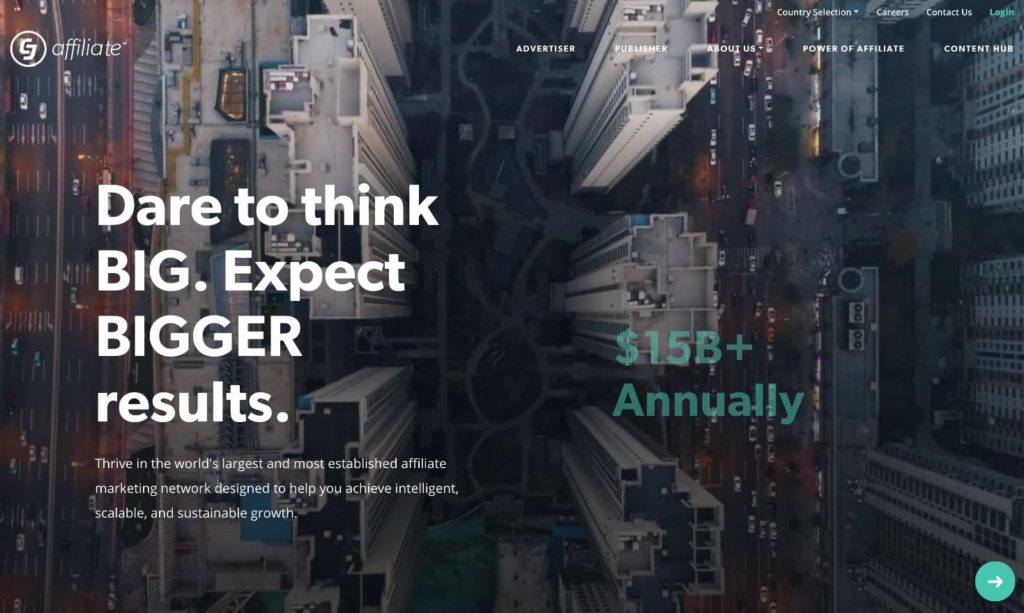The image appears to be the landing page of a company website, designed with a modern and engaging layout. Dominating the left side of the graphic is a bold and motivational slogan, "Dare to Think Big, Expect Bigger Results," drawing immediate attention. On the right side, there's a prominent figure, "15 billion+ annually," accompanied by a dollar sign, indicating this is in US dollars. This impressive statistic is linked to the statement, "Thrive in the world's largest and most established affiliate marketing network, designed to help you achieve intelligent, scalable, and sustainable growth."

In the top left corner, the word "Affiliate" is displayed next to a logo, although the logo is not clearly identified. Below this, a navigation menu includes links labeled "Advertiser," "Publisher," "About Us," "Power of Affiliate," and "Content Hub." Just above this menu, additional links are present, providing options like "Country Selection," "Careers," "Contact Us," and "Login."

Behind all these elements is a captivating aerial photograph taken from the top down, likely by a drone or helicopter, showcasing an urban landscape filled with high-rise buildings. The overall design successfully integrates text and imagery to create an impressive and informative landing page.